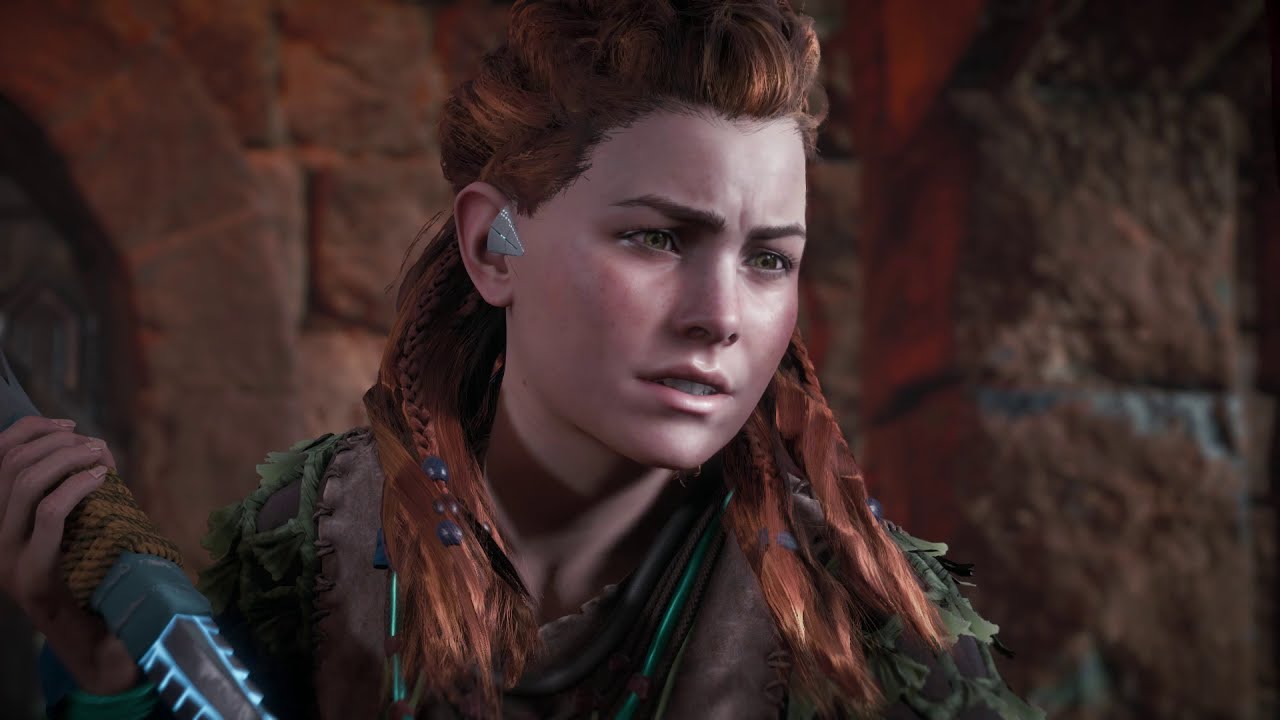This image is from a well-known video game, possibly named Lost Horizon or something similarly familiar. It features a close-up of the main character, a young woman with long red hair tied back and draping over her shoulders. Her hair includes braids adorned with dark blue beads. She has a triangular metallic piece near her right ear that stands out against her raggedy tunic made of leather and green fabric. Her hazel eyes convey concern or pain as she looks to her side. She is holding a glowing blue dagger-like weapon in her right hand. The scene appears to be computer-generated with a touch of realism, though some angles seem slightly off. The background shows a blurred, reddish brick wall, suggesting this is from a cinematic moment in the game.